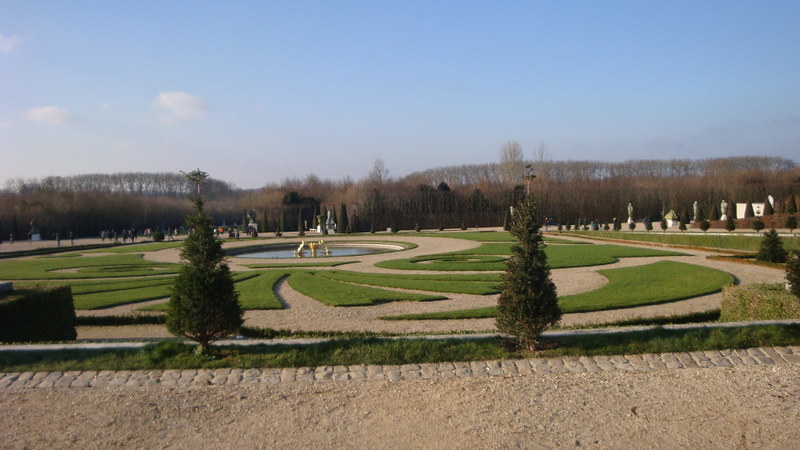This outdoor photo, likely taken in the afternoon, showcases a detailed park scene during what appears to be late autumn or early winter. The foreground features a gravelly and rocky area bordered by a brown cement wall or stone pathway. Just beyond this, there's a grassy section with evenly spaced pine trees and shrubs on either side. Various curved concrete sidewalks interspersed with intricately cut strips of grass and sand lead to the focal point—a circular fountain in the center. The fountain, which has a gold centerpiece, appears to be inactive at the moment. Surrounding the fountain are people leisurely walking and observing the surroundings. In the distance to the right, additional statues emerge from behind barriers, accompanied by a dense arrangement of trees. To the left, more statues and a group of people can be seen entering the area. The background is filled with dry, barren trees and mountains against a blue sky, all contributing to the park's serene and well-maintained atmosphere.